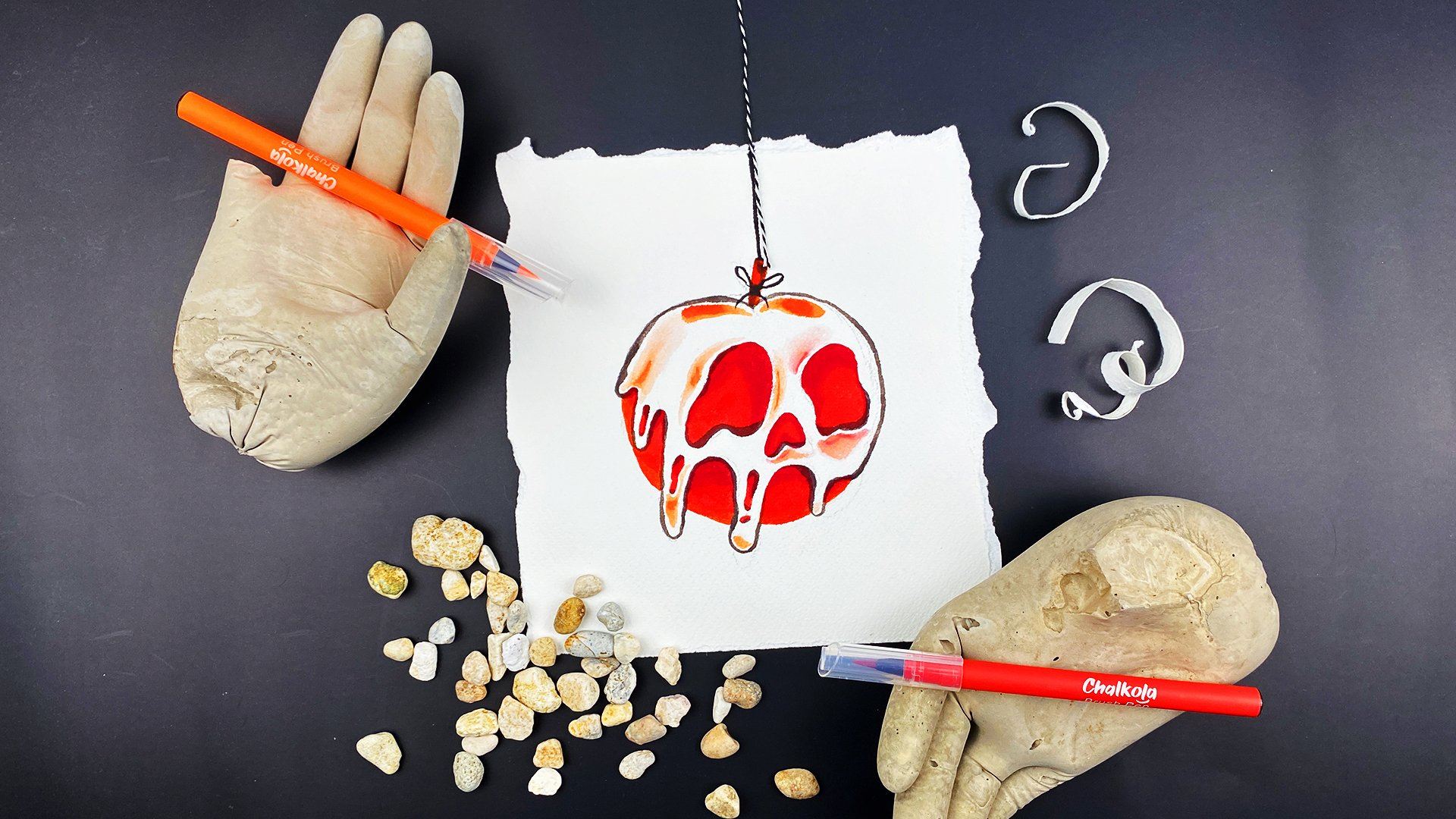The image showcases an intriguing art installation set against a navy blue background. Dominating the center is a jagged, square piece of white paper featuring a red-orange apple tied to a string extending upwards. The apple is partially covered in a white, skull-like ooze that drips elegantly, revealing gaps of the apple's surface. To the right of this central piece lies a cluster of curled, white paper strips. On the left, an assortment of pale-colored pebbles in shades of yellow, blue, and pink adds texture. In the upper left corner, a plastic glove, filled with some material and missing its pinky finger, holds an orange marker labeled "Chocola" with its palm facing up. In the upper right corner, another gloved or possibly plaster hand, thumb removed, grips a red marker with a clear cap. The overall composition, fixed against the dark blue backdrop, evokes a surreal, contemporary artistic theme.